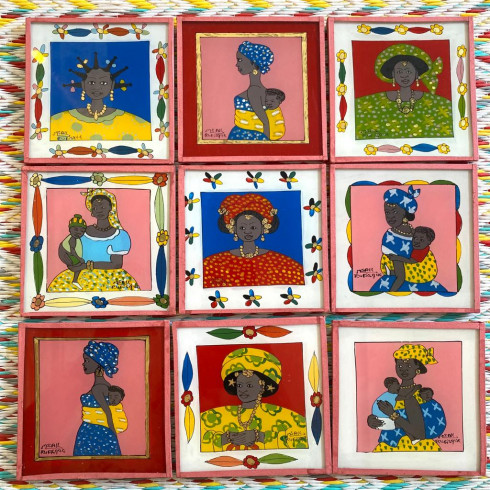The image is a vibrant and detailed collage of nine cartoon drawings, each set within a pink wooden frame arranged in a 3x3 grid. The entire collage is surrounded by a white border adorned with a colorful tribal pattern featuring yellow, green, and red designs, giving it a distinct ethnic flair. Each drawing depicts an African or African-American woman with dark skin, styled in traditional clothing and various head coverings. 

In the top left square, the woman is wearing a yellow shirt, her spiky hair radiating outward like needles or a porcupine. The second square features her in a blue gown, adorned with a head wrap, and carrying a child on her back in a traditional fabric wrap. In the third square, she dons a wide green dotted dress paired with a matching head wrap. 

The fourth image shows the woman holding a child to her right, whereas the fifth square has her in a red version of the dress seen in the third image. The sixth image repeats the blue dress with the child attached to her back again, similar to the second square.

The seventh image mirrors the second except her earrings are different. In the eighth square, she wears a yellow and green version of the wide dress from the third image. Finally, the ninth square depicts the woman placing a child on her front while carrying another child on her back, showcasing a rich and dynamic depiction of traditional childcare.